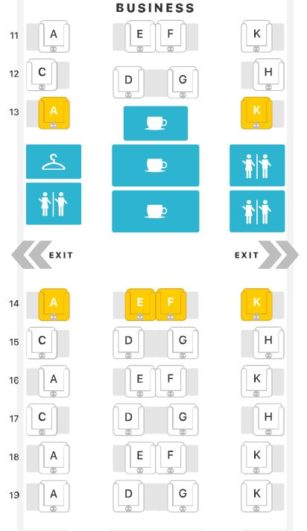The image appears to be an annotated floor plan of a business establishment, possibly a coffee shop, illustrated in a stylized, key-like format. At the top center of the image, the word "BUSINESS" is prominently displayed in bold, black, capital letters, center-aligned. Below "BUSINESS," the letters "E" and "F" are featured within square-shaped areas that appear to be designated seating sections, surrounded by bench-like seating arrangements. These sections are color-coded, with some areas in white and others in yellow.

On the left-hand side of the image, a vertical series of numbers is displayed, starting from 11 and sequentially continuing through to 19, which may designate different sections or tables. In the central area, there are several blue boxes. Three of these boxes contain icons of coffee cups, suggesting they are coffee stations or seating areas catering to coffee service. Another blue box, featuring a clothes hanger icon, may represent a coat check or storage area. Overall, this detailed layout provides a clear and organized overview of the business's seating and service arrangement.